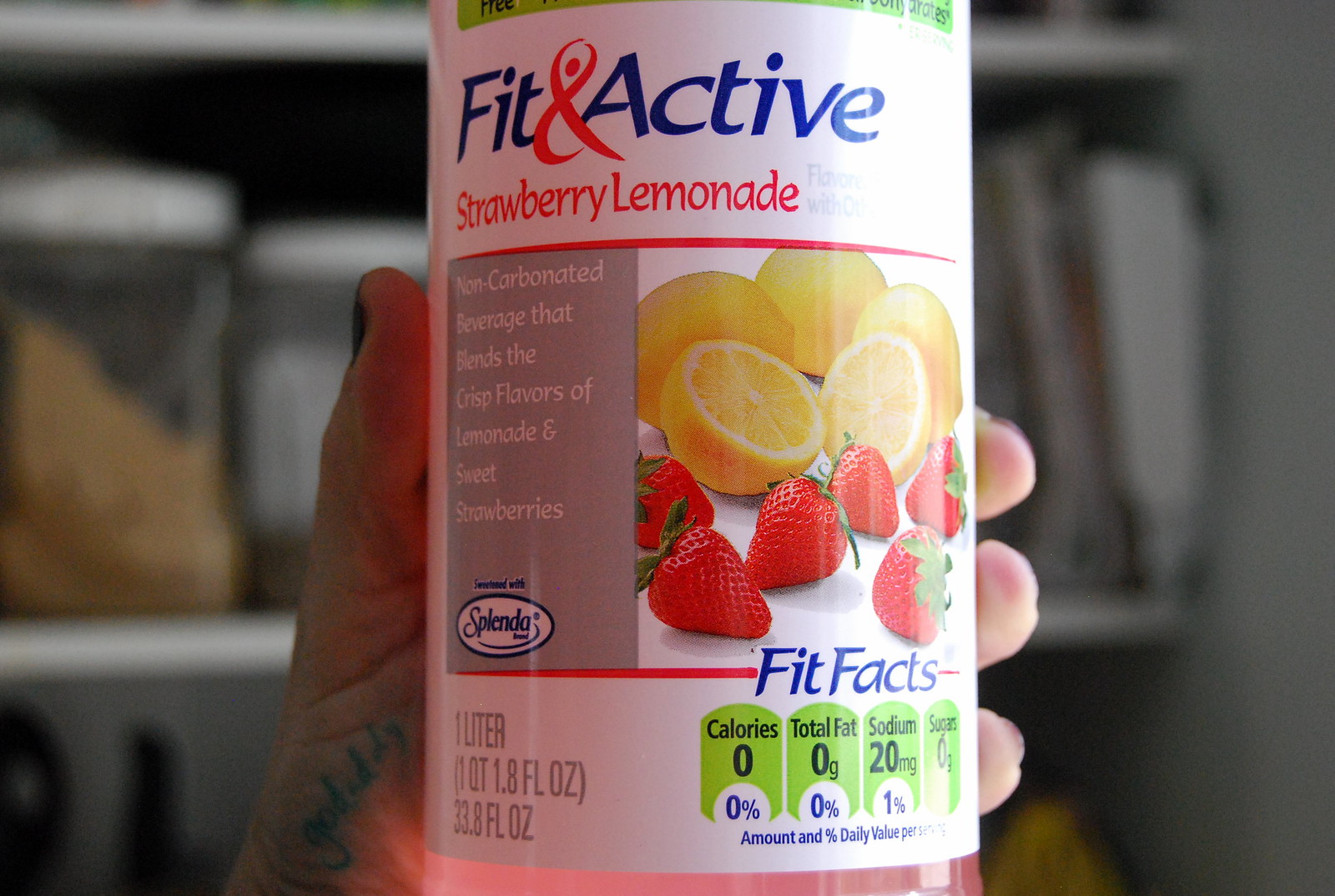The image features a hand holding a bottle of strawberry lemonade juice from the brand Fit & Active. The juice is a non-carbonated beverage that combines the crisp flavors of lemonade with sweet strawberries and is sweetened with Splenda. The bottle is labeled as one liter, which is equivalent to 33.8 fluid ounces. 

The front of the bottle showcases detailed nutritional information, highlighting zero calories, zero total fat, 20 milligrams of sodium, and zero grams of sugars per serving. 

To the right of the label, the imagery includes three whole lemons and one lemon cut in half, as well as several whole strawberries, emphasizing the natural ingredients used in the beverage. 

The hand holding the bottle is adorned with dark burgundy or black nail polish and has a distinctive tattoo that reads "go daddy". The background and focus on the hand add a personal touch to the image.